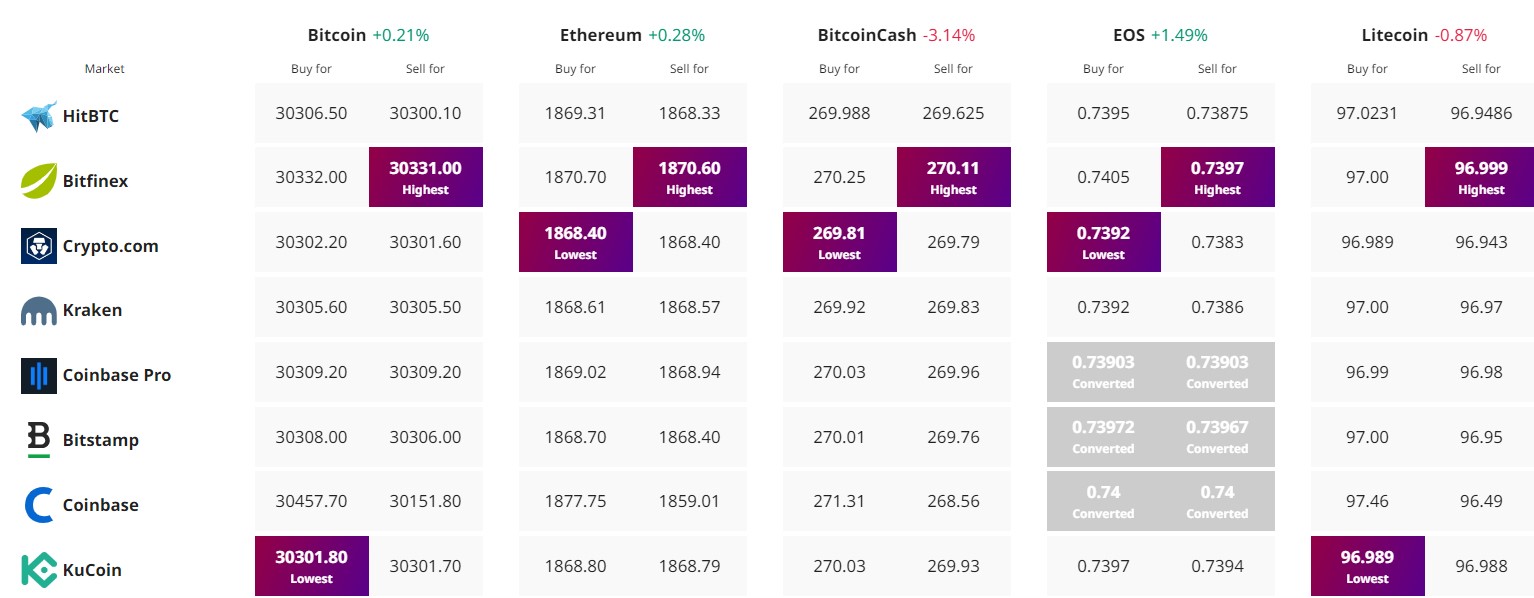A detailed image of a cryptocurrency trading page showcases a variety of digital currencies such as Bitcoin, Ethereum, Bitcoin Cash, EOS, and Litecoin. The page features multiple exchanges including HBTC, Bitfinex, Crypto.com, Kraken, Coinbase Pro, Bitstamp, Coinbase, and KuCoin. The trading chart prominently displays the prices for buying and selling these cryptocurrencies. On the left side, the section marked "Buy" lists specific prices, which correspond to prices in the "Sell" section on the right. Several areas within the chart are represented with burgundy and purple-colored rectangles, highlighting important data points. In particular, the EOS section shows a positive change of +1.49%. Below this, there are three boxes indicating conversion values with a sample figure of 0.73903, labeled as "converted." The figures on both the right and left sides of these sections appear to be balanced, visually emphasizing the conversion data's accuracy.